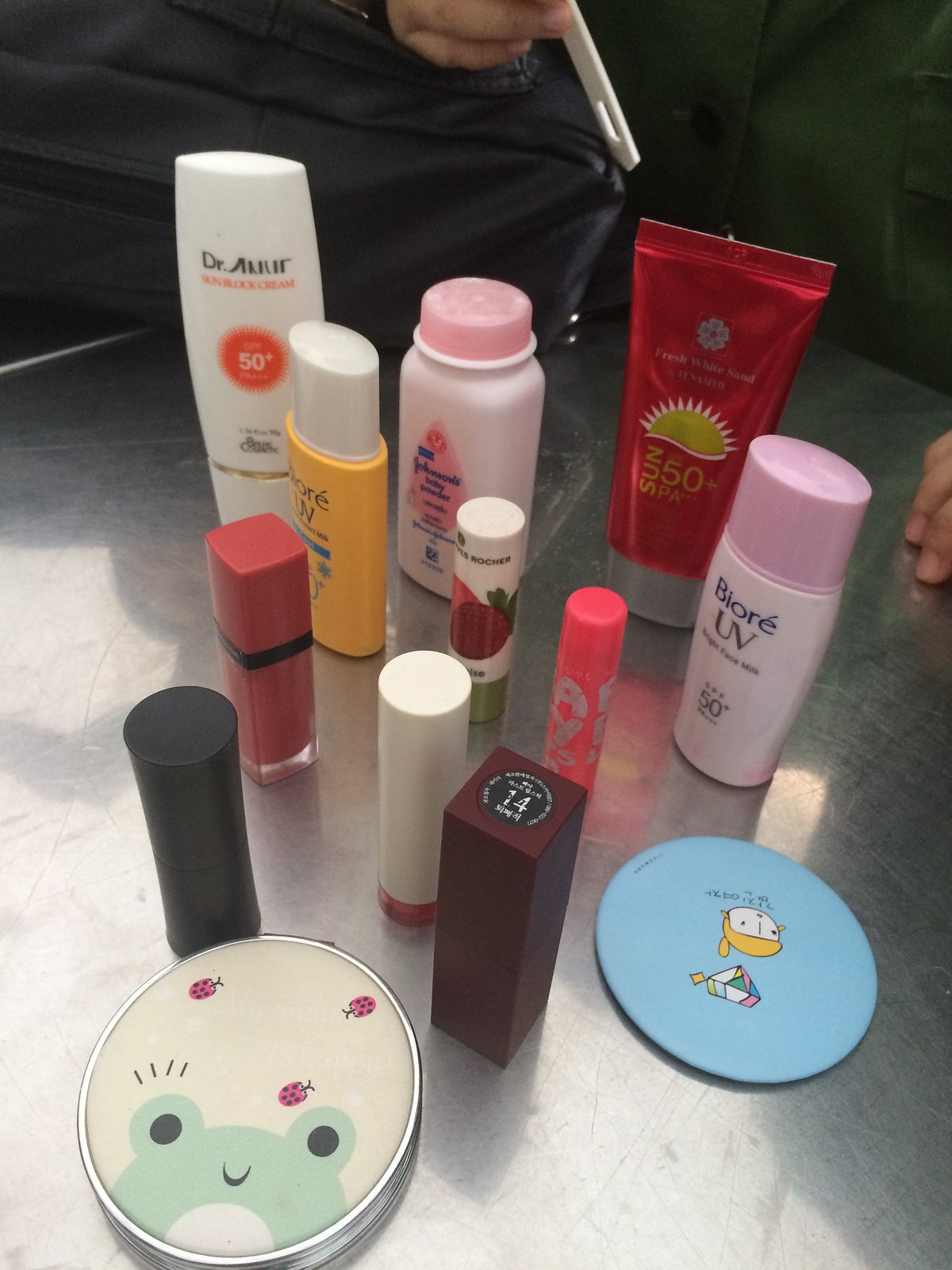Arrayed on a sleek, metallic-looking tabletop are an assortment of beauty products, creating a vibrant display of various shapes and colors. On the left side of the frame stands a white plastic bottle prominently marked with "SPF 50+" within a bold red circle. Adjacent to it, there is a bright yellow bottle with a white cap, labeled "BRUV." In front of the yellow bottle, a striking red tube of lipstick catches the eye, its square body elegantly decorated with a black design. Nearby, we spot another tube resembling lip balm, featuring a green cap and adorned with fruit illustrations on its front. 

Adding to the mix is a bottle of Johnson's powder, distinguished by its pink cap and square shape. A shiny, deep red sunscreen container with "Sun 50+" emblazoned on it asserts its presence among the array. Finally, a Biore UV container with a light pink cap and a pristine white body completes the orderly yet lively collection. Sprinkled throughout the scene, additional lipsticks and beauty items populate the tabletop, inviting a closer look at the variety of personal care products displayed.